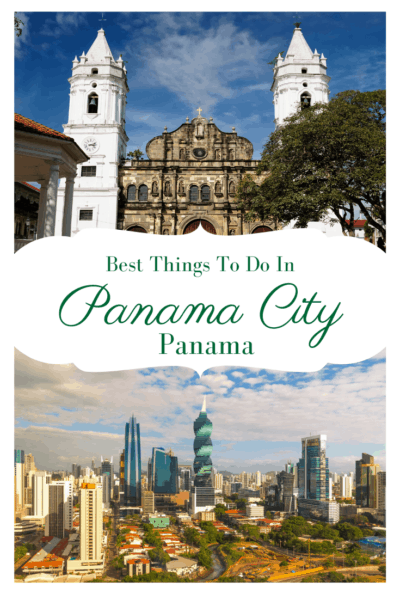The image consists of two separate photographs stacked vertically, separated by a wavy, cloud-shaped banner that is white. In green script, the banner reads, "Best things to do in Panama City." The word "Panama" appears in a smaller script underneath.

The top photograph depicts a clear sky with sparse, loose clouds. Prominently featured is a cathedral-like structure with two pointed towers flanking a central building. The overall structure is white with a middle section that appears brown and features numerous windows. To the right, a tall, bushy tree with lush green leaves adds to the scenery.

The bottom photograph, placed below the banner, displays a sky with more clouds than the top picture. In this image, a series of uniquely shaped buildings draw the eye. Central to the picture is a structure that resembles a twirled lollipop stick, with segments in light green, teal, and a white tip, evocative of an upside-down spiral design. The left side of the photograph features beige and white buildings, while the right side displays green-colored buildings, likely reflecting the tint from their glass panels, interspersed with verdant trees.